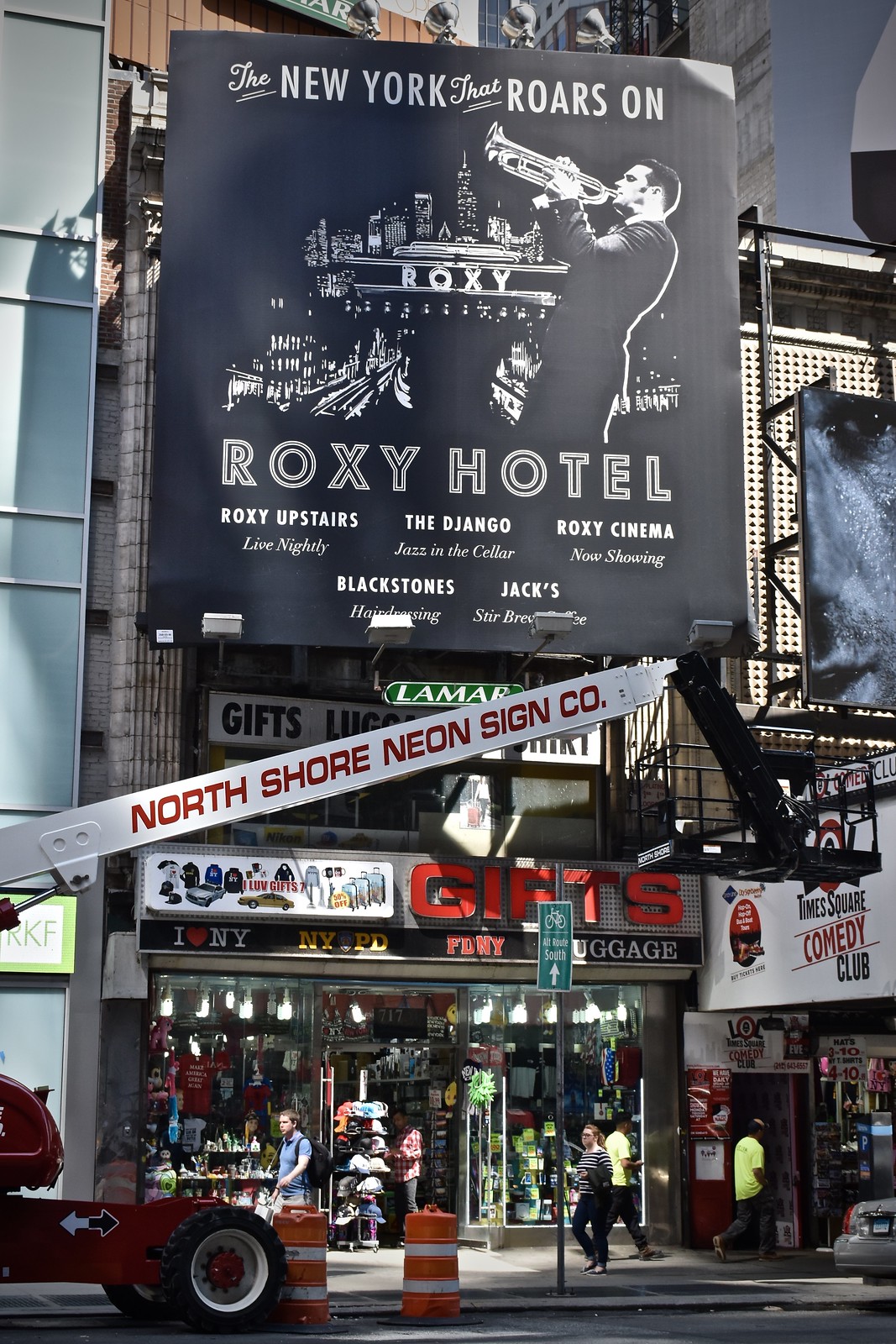The photograph depicts a busy New York City street scene taken during the daytime. From our vantage point across the street, we see a storefront and multiple advertisements on a building directly ahead. In the lower left-hand corner, the back end of a red crane with "North Shore Neon Sign Co." in bold red letters on a white bar is visible. The crane extends diagonally from the bottom left towards the upper right. Nearby, two orange and white barrels are positioned behind the crane, while pedestrians navigate the sidewalk around it. The store's windows showcase various clothing items, hats, and tourist trinkets, with signage above reading "I ♥ New York," "NYPD," "FDNY," and "luggage". To the right of the crane's boom, a white banner advertises the "Times Square Comedy Club". Above this setup, a large black billboard announces "The New York that roars on," featuring an image of a man playing a trumpet. Beneath this, the advertisement lists several venues: "Roxy Hotel," "Roxy Upstairs," "The Django," "Roxy Cinema," "Blackstones," and "Jacks." The scene captures the essence of a bustling metropolis filled with lively commerce and vibrant advertisements.